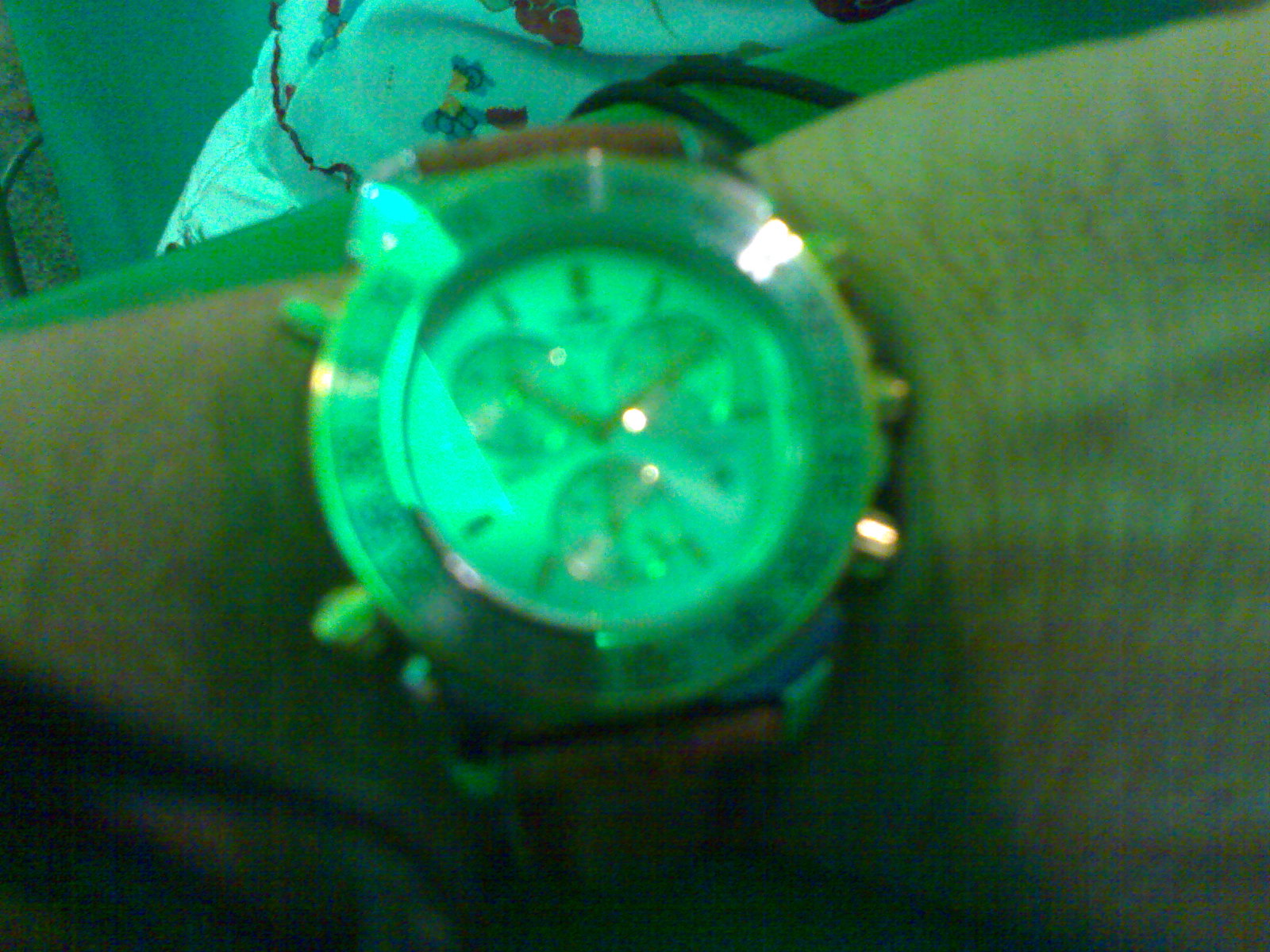The image features a close-up of a person's wrist adorned with a gold-faced watch. The watch face, about six inches in both width and height, is illuminated by a striking green light, which enhances its visibility. The face of the watch, surrounded by a brown leather band, is positioned dead center in the photo. The face itself is white and includes three smaller circles and gold watch hands that point towards the left and right, although the image is a bit blurry due to the proximity to the camera. The person's arm, which is rather hairy, shows faint, black hairs along the skin. In the background, there appears to be a white sheet or pillow with a blue print, possibly featuring cartoon characters, adding a playful element to the scene.